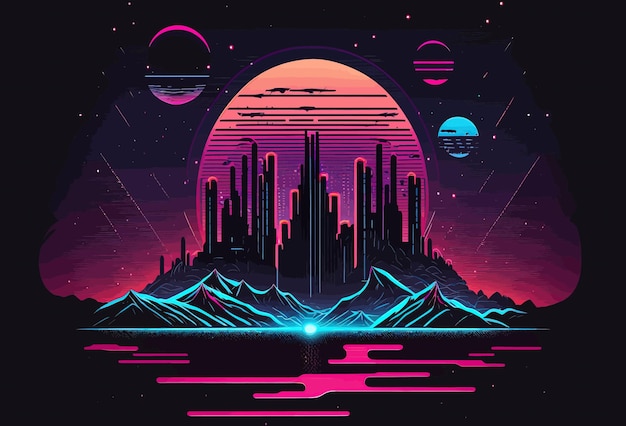This artwork, reminiscent of neon design aesthetics, vividly showcases a futuristic cityscape with an array of bright, striking colors set against a black backdrop. Dominating the center is a large, roundish form that expands from a narrow top to a broader bottom, enclosed by a flat base. The scene within this form depicts tall, pinkish-purple skyscrapers emerging from behind blue-outlined, black mountains, with the peaks tinged in hues of pink and purple. A bright white-blue light stretches horizontally across the picture, just below the mountains. In the sky, stars and a mix of celestial bodies punctuate the backdrop, including one prominent circle on the left and two on the right, colored in shades of purple and pink. This blend creates a dynamic and immersive environment that feels like a snapshot from a sci-fi movie, inviting viewers to explore the enigmatic city and its futuristic possibilities. Additionally, asymmetrical pink lines interspersed at the bottom add an abstract touch, enhancing the artistic flair.